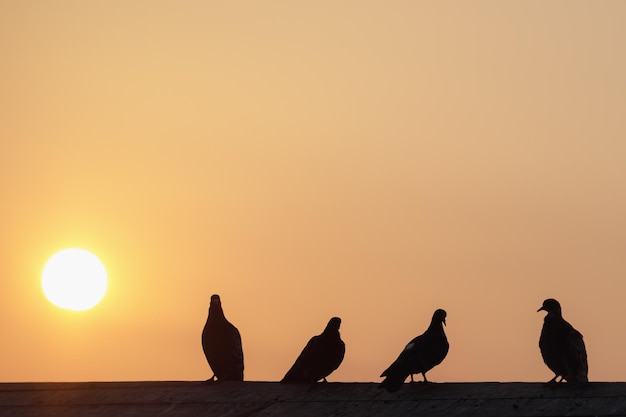The photograph captures an exquisite sunset scene with the sky painted in shades of dark orange, peachy pink, yellow, and hints of brown. A blinding white sun is nestled in the lower left corner, casting a rich glow across the entire image. Against this radiant backdrop, a long, dark, slanted roof occupies the bottom portion of the frame. Perched atop the roof are four black silhouetted birds. From left to right, the first bird is facing forward, the second bird appears to be facing backward, the third bird is facing right with its legs clearly visible, and the fourth bird, positioned at the far right, is facing left. The harmonious blend of colors and the composition of the silhouetted birds against the sunset sky brilliantly showcase the beauty of nature.